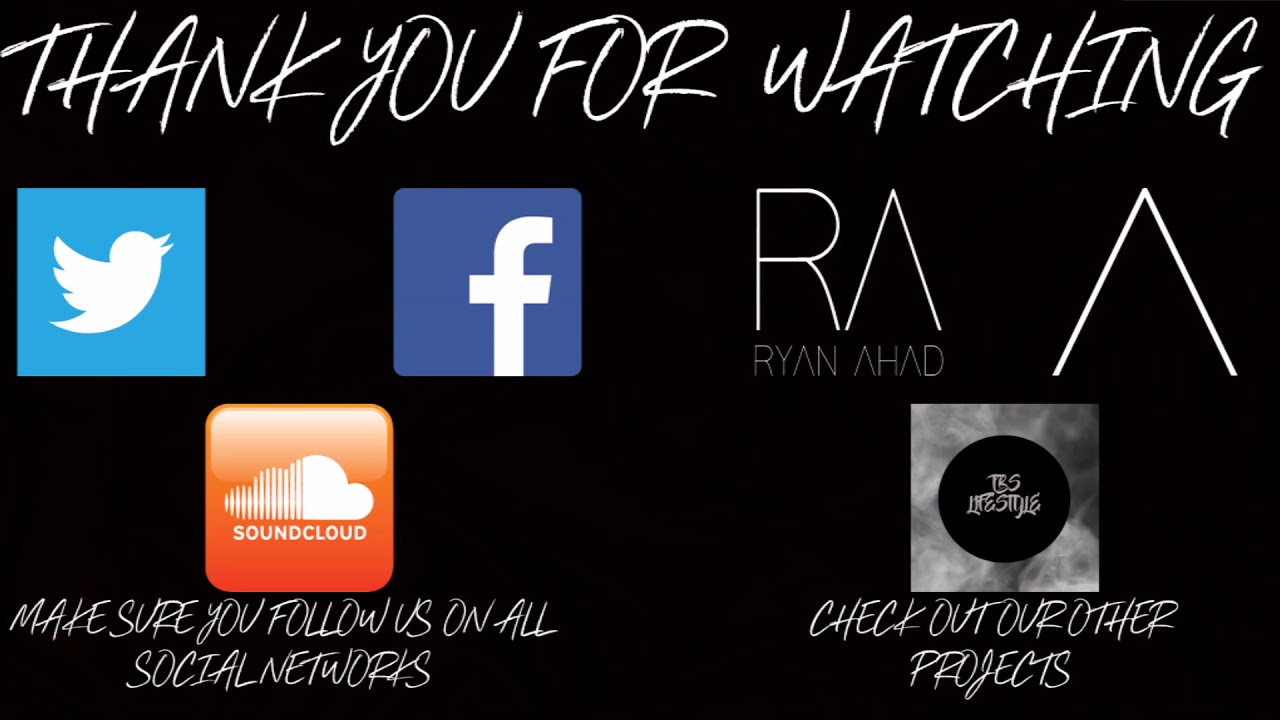The image has a solid black background with white text prominently saying "THANK YOU FOR WATCHING" at the top. Below this, on the left side, there are square logos for Twitter, Facebook, and a more 3D-effect SoundCloud logo. Directly below these logos, in white, all-caps text, it states, "MAKE SURE YOU FOLLOW US ON ALL SOCIAL NETWORKS." On the right side, under the "THANK YOU FOR WATCHING" text, there is a stylized logo for Ryan Ahead, with a capital "R" and a triangular "A." Adjacent to this is the name "R.A. Ryan Ahad," followed by a small carrot symbol. Underneath, there is a logo featuring "TRS Wrestling" and another enigmatic logo with the text "TBS Lifestyle," which consists of a black circle and a gray, smoky square. In the bottom right corner, in white text, it says, "CHECK OUT OUR OTHER PROJECTS."